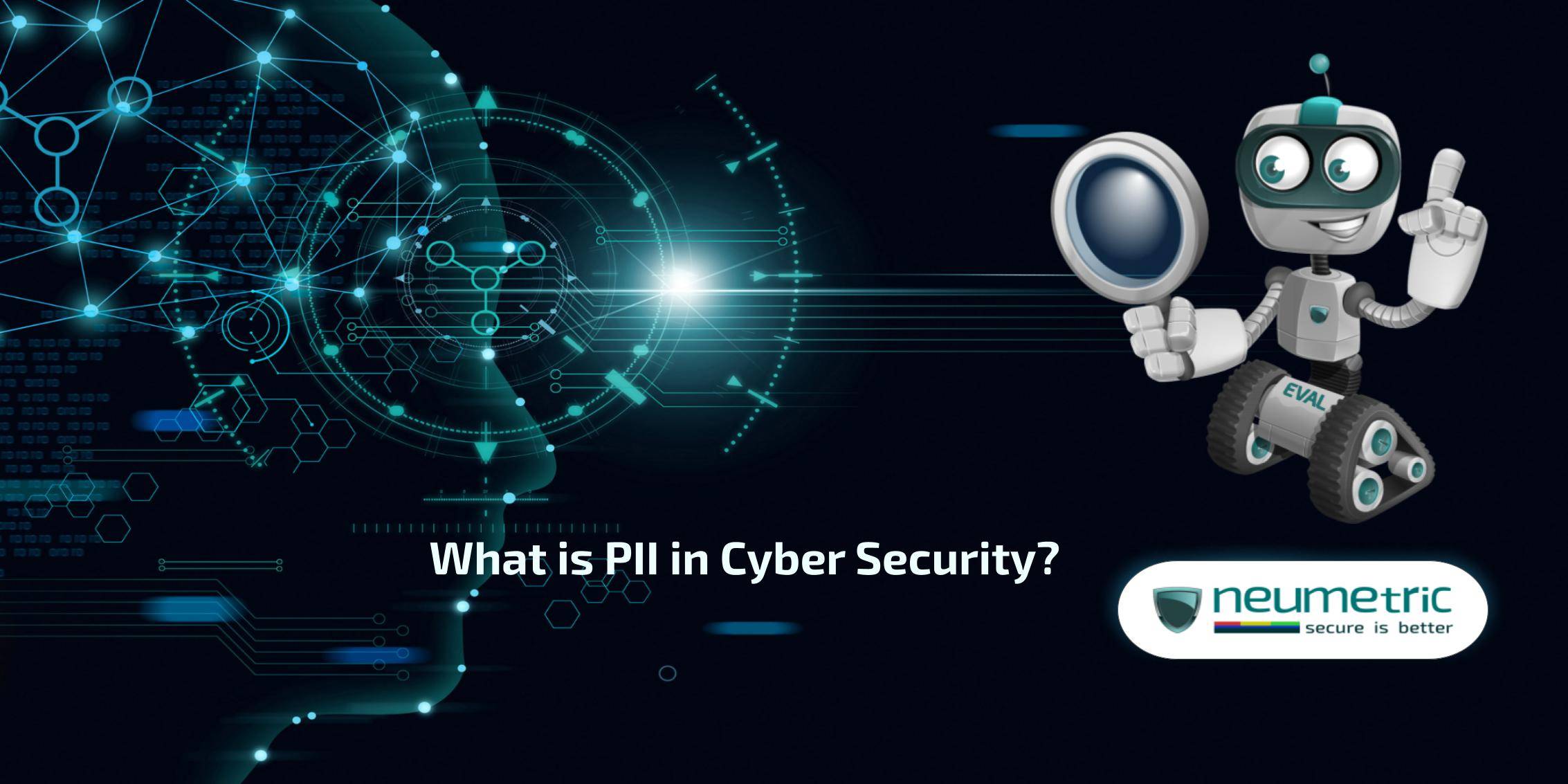This is an advertisement for the cybersecurity company Numetric (N-E-U-M-E-T-R-I-C) with a tagline "Secure is better." The background is a deep navy blue, almost black. The left side of the image features an intricate design combining an anatomical profile of a human head with technical drawings. Superimposed on the head are glowing blue and white sprockets, gears, and chemical formulation shapes, creating a sense of a complex, interconnected system. 

On the right side of the image, a friendly, playful robot character, reminiscent of WALL-E, captures attention. This 3D-rendered robot has silver body with tank-like caterpillar tracks instead of wheels, googly eyes with green accents, and a surprised, yet friendly expression. It has a green stripe down the middle of its head and one blue antenna. The robot is holding a magnifying glass in its right hand, pointed towards the left side of the image, while its left hand has a pointer finger raised as if making a point. 

Above the robot, the tagline "What is PII in cybersecurity?" is displayed in bold white lettering. At the bottom right corner of the image, there is an oblong white oval containing the company's name, "Numetric," in green letters, followed by the slogan "Secure is better."